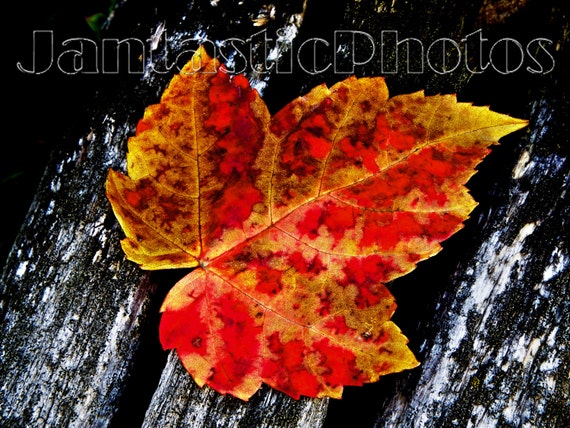The image captures a vibrant leaf in the midst of autumn, displaying a captivating gradient of yellow, orange, and red, indicative of its seasonal transition. The leaf, which resembles a maple leaf with its characteristic three-lobed structure, is prominently placed atop a background of aged, weathered wood. The wood surface features diagonal striations running from the lower left to the upper right and exhibits a mossy texture with varying shades of dark blotches, enhancing the rustic aesthetic. At the top of the image, semi-transparent, hollow white lettering spells out "Jantastic Photos," adding a subtle yet noticeable watermark that blends harmoniously with the natural elements. The contrast between the vivid hues of the leaf and the subdued, grayish tones of the wood makes the leaf's colors exceptionally striking, creating a vivid focal point within the composition.